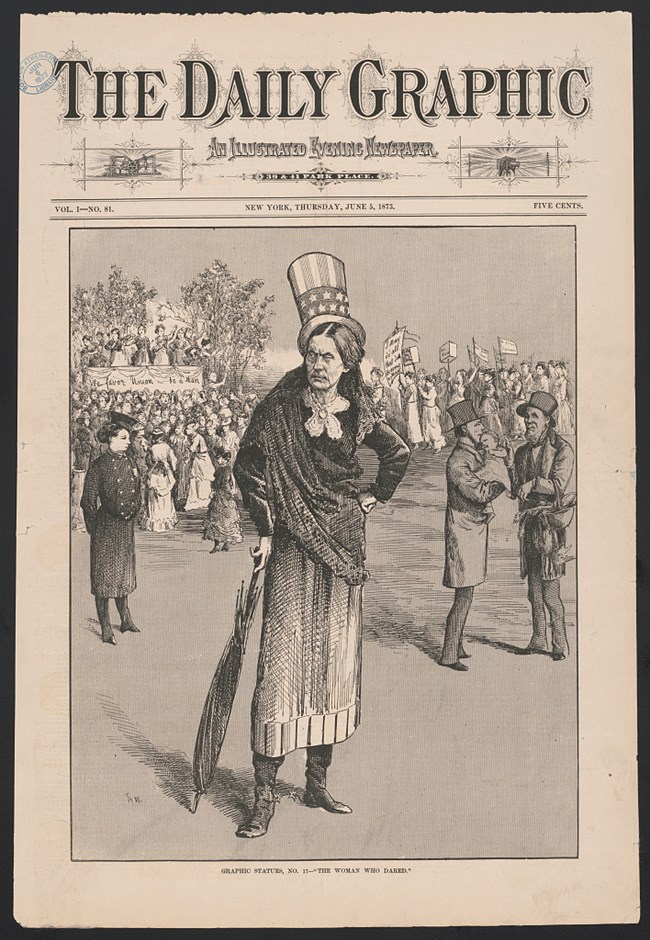This image features a vintage page from "The Daily Graphic," an illustrated newspaper, under a light pinkish beige background often associated with aged paper. The publication details at the top include "The Daily Graphic" in large black letters, followed by "An Illustrated Evening Newspaper." It specifies Volume 1, Number 81, New York, Thursday, June 5, 1873, priced at five cents. 

Centered on the page is a detailed black and white illustration of a woman donning an Uncle Sam hat adorned with stars and stripes. She wears a long dress that reaches her ankles, coupled with boots and a shawl draped over her right shoulder. A decorative pin or bow fastens at her throat, crossing at the chest. An umbrella in her right hand points downward to the ground, resembling a walking stick. She stands with one hand on her hip, gazing to her right.

The backdrop of the drawing is bustling with action, featuring multiple individuals carrying flags and signs, indicating a march or protest. The scene includes a policewoman in uniform positioned near the left center and two gentlemen in top hats and long coats engaged in conversation on the right. Additionally, women appear on a stage in the upper left of the image, with trees and more marchers in the background, suggesting an eventful gathering.